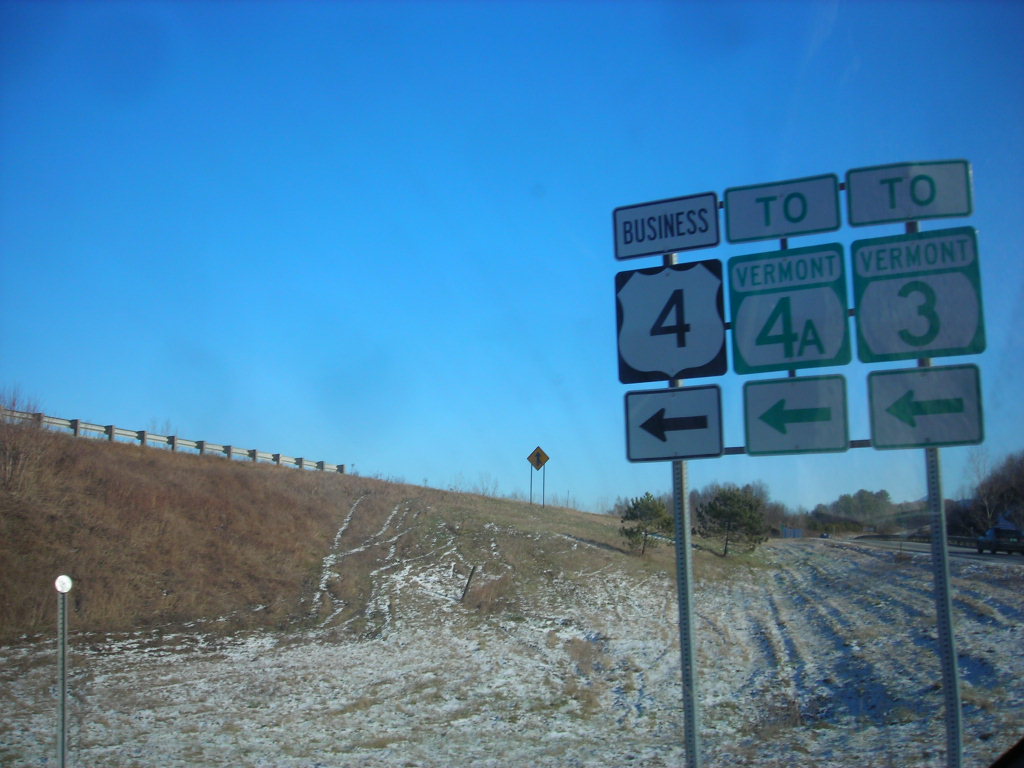This daytime photograph captures a scene under a brilliantly blue sky. In the foreground, a hill slopes upward to the left, partially covered by thin layers of snow. Sparse brush is visible on the hillside, creating a textural contrast with the snow. At the crest of the hill, a street with a guard railing can be seen, emphasizing the elevation. 

Prominently rising from the bottom right corner is a large street sign with three distinct panels. The leftmost sign directs toward "Business 4" with an arrow indicating a left turn. The central sign points travelers towards "Vermont 4A," also with a left-turn arrow. The rightmost sign guides to "Vermont 3" with a similar left-arrow. This combination of natural and man-made elements creates a dynamic and informative landscape.